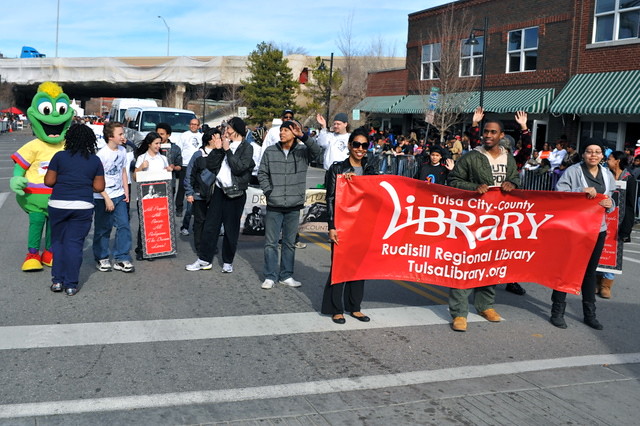This image depicts a vibrant parade marching down a city street in Tulsa, Oklahoma. In the background, a brick building with a green and white awning is visible, along with an overpass and several vehicles, including a van. The foreground features three African American individuals holding a prominent red banner with white lettering that reads "Tulsa City-County Library, Rudisill Regional Library, Tulsalibrary.org." To the left, a lively green mascot with a yellow mohawk, wearing a yellow t-shirt and yellow and red shoes, adds to the festive atmosphere. The scene is set near the intersection, possibly around Greenwood Archer and Pine, with a visible crosswalk at the bottom of the image. The sun casts long shadows, suggesting it's late in the afternoon. Enthusiastic spectators line the street, contributing to the lively mood of the event.